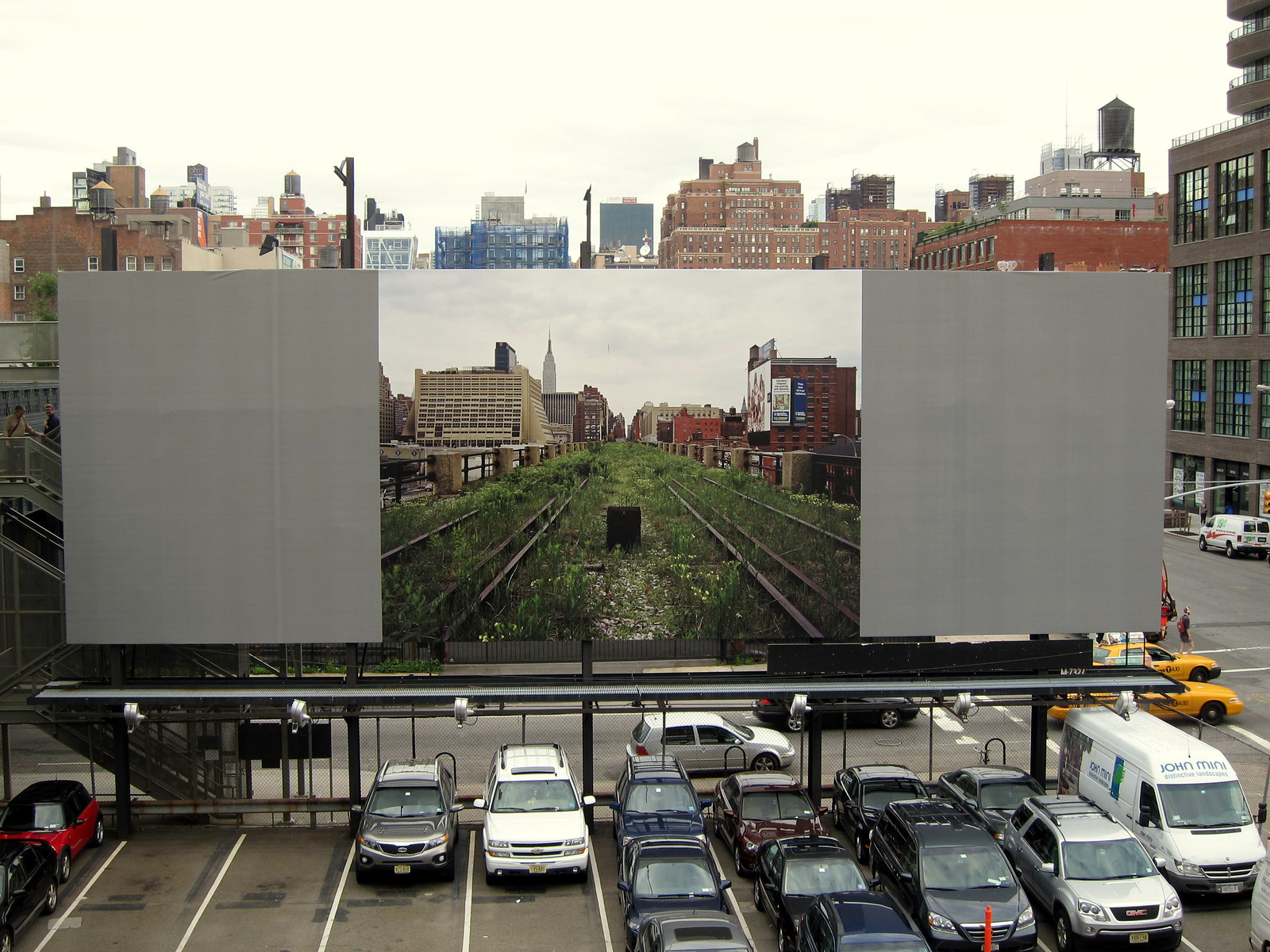A panoramic cityscape unfolds under a foreboding sky, showcasing a variety of towering buildings cloaked in hues of brown, red, blue, and gray. Dominating the center of the frame is a massive structure that appears to be either a billboard or an outdoor theater screen. This screen features an image of train tracks that have been overtaken by grass, flanked by buildings on both sides, creating a striking visual contrast. On either side of this central structure, dark gray facades add to the urban motif. Below, approximately 10 to 15 cars and vans of various models are neatly parked within white-lined spaces on a gray asphalt surface, adding an element of everyday life to this urban tableau.